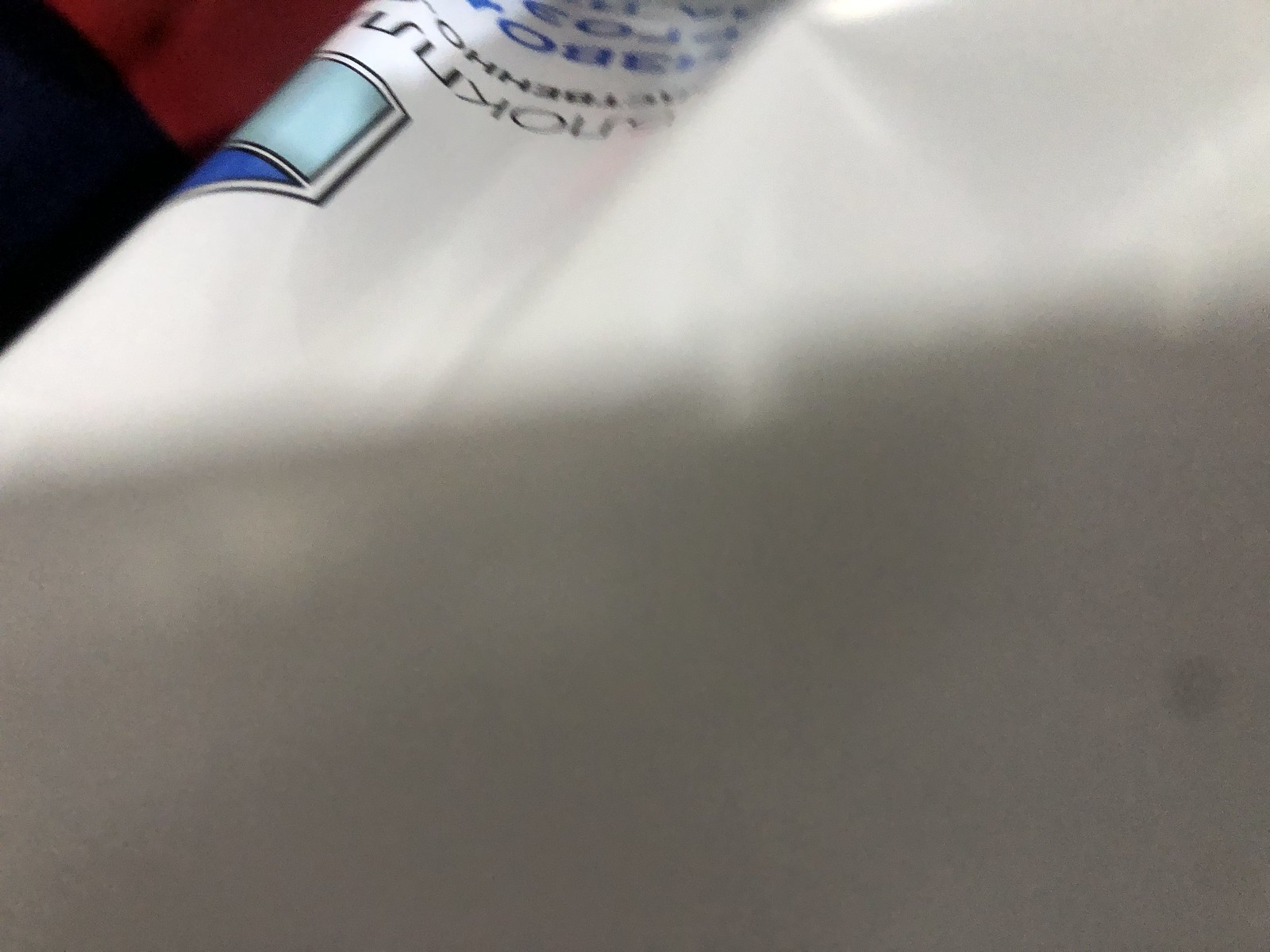The image features a close-up view of the upper left corner of a white piece of paper. Behind the paper, part of a red and blue fabric is visible, with the red fabric located in the upper right section and the blue fabric, which may be denim or a shirt, in the lower left section. On the white piece of paper, in its upper left corner, there is a blue and sky blue polygon, distinctly separated by a white barrier outlined in black. Above this polygon, there is a line of black text, and further above that, blue text.